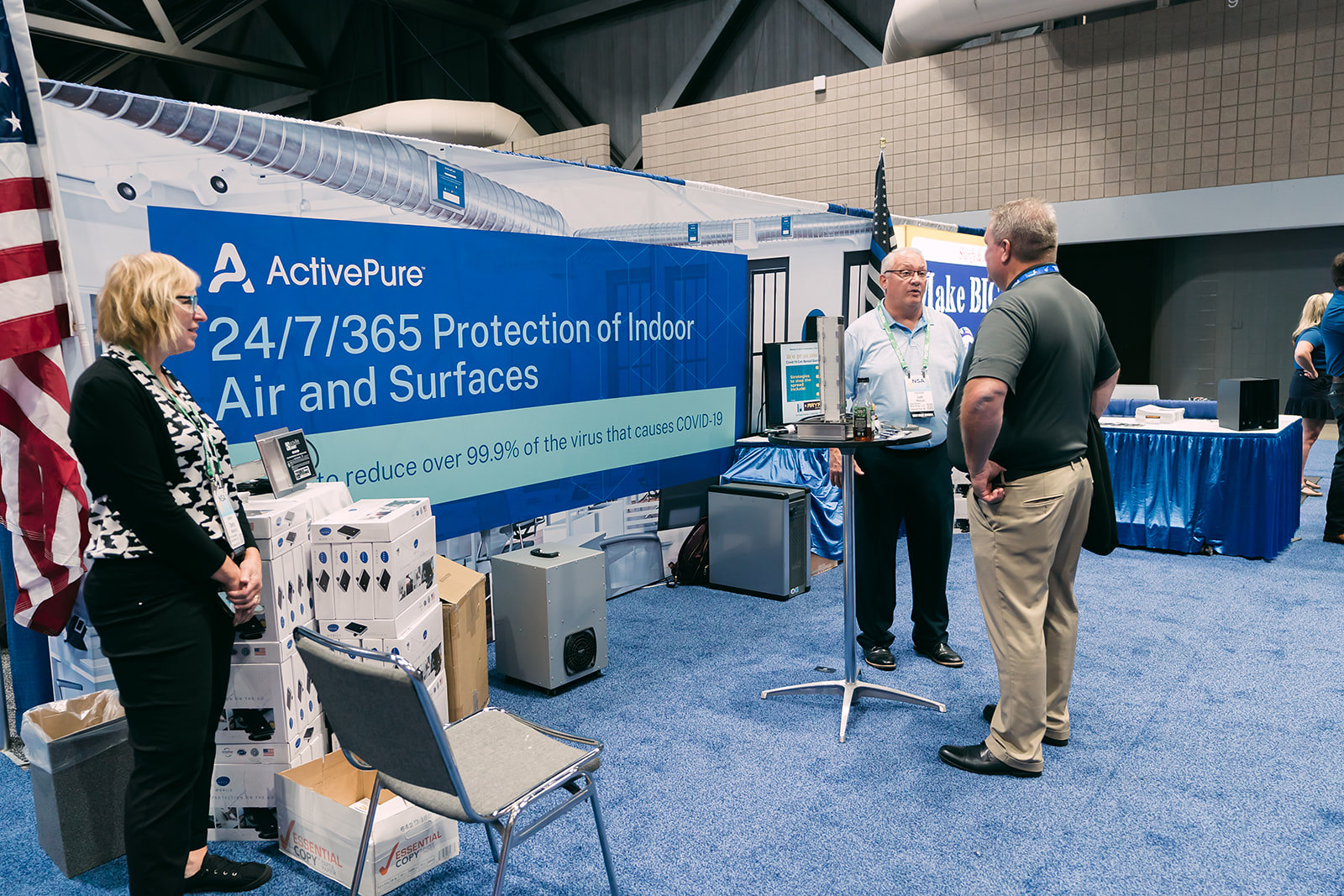The image is a rectangular photograph taken indoors, likely at a conference or an exhibition in an older stadium. The focal point is a booth featuring Active Pure, a brand promoting its product that claims 24-7, 365 days of protection for indoor air and surfaces, and reducing over 99.9% of the virus that causes COVID-19. A large blue banner with white and light blue text displaying this information is prominently seen in the background, flanked by two American flags.

In the foreground, on the right side of a plush blue carpet, two older men are engaged in conversation. The man closest to the camera is slightly taller, with graying hair, and is dressed in a gray short-sleeved shirt, khaki pants, and black dress shoes. His conversation partner, also with graying hair and glasses, is wearing a short-sleeved blue polo shirt, black pants, and black dress shoes. A small waist-high circular table stands between them.

On the left side of the image, a woman of Caucasian descent with blonde hair and glasses observes the scene. She is wearing a long-sleeved black shirt, black pants, and a white vest with a black print, and she too has a lanyard around her neck. Behind her is a stack of white boxes, an empty chair, and one of the American flags. Above the scene, the open ceiling reveals rafters, beams, and ductwork, reinforcing the indoor stadium setting.

Additionally, the booth area includes more tables, scattered chairs, a garbage can, and other items, contributing to the bustling atmosphere of the conference.